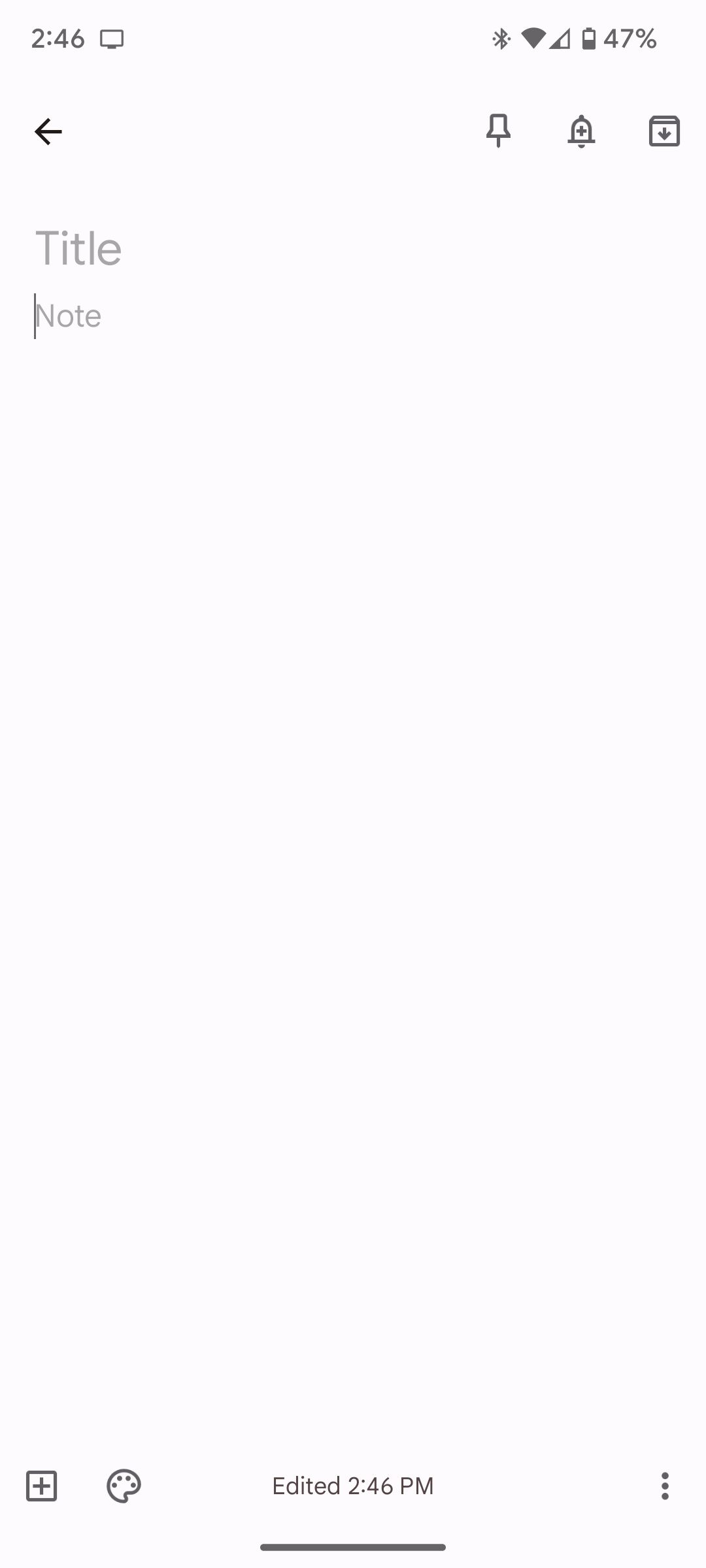The image depicts a screenshot from an Android device taken at 2:46 PM. In the notification area at the top of the screen, there is an unfamiliar icon resembling a rectangle with a small symbol underneath, potentially indicating a message or another notification. Nearby, the status area displays familiar symbols: Bluetooth connectivity, Wi-Fi signal strength, and a notably weak mobile data connection represented by a partially filled triangle. The battery level is at 47%.

The primary focus of the screenshot is a note-taking app interface. At the top left corner, there is a return arrow, while the top right corner houses a pushpin, a bell, and a calendar icon. The main body of the app features two gray placeholder texts labeled "Title" and "Note," with the cursor positioned at the start of the "Note" field. The majority of the screen is occupied by an empty space for typing.

At the bottom of the screen, there are additional icons for adding content: a plus sign, a square, an artist palette, along with text that indicates the note was edited at 2:46 PM, and a three-dot menu for more options.